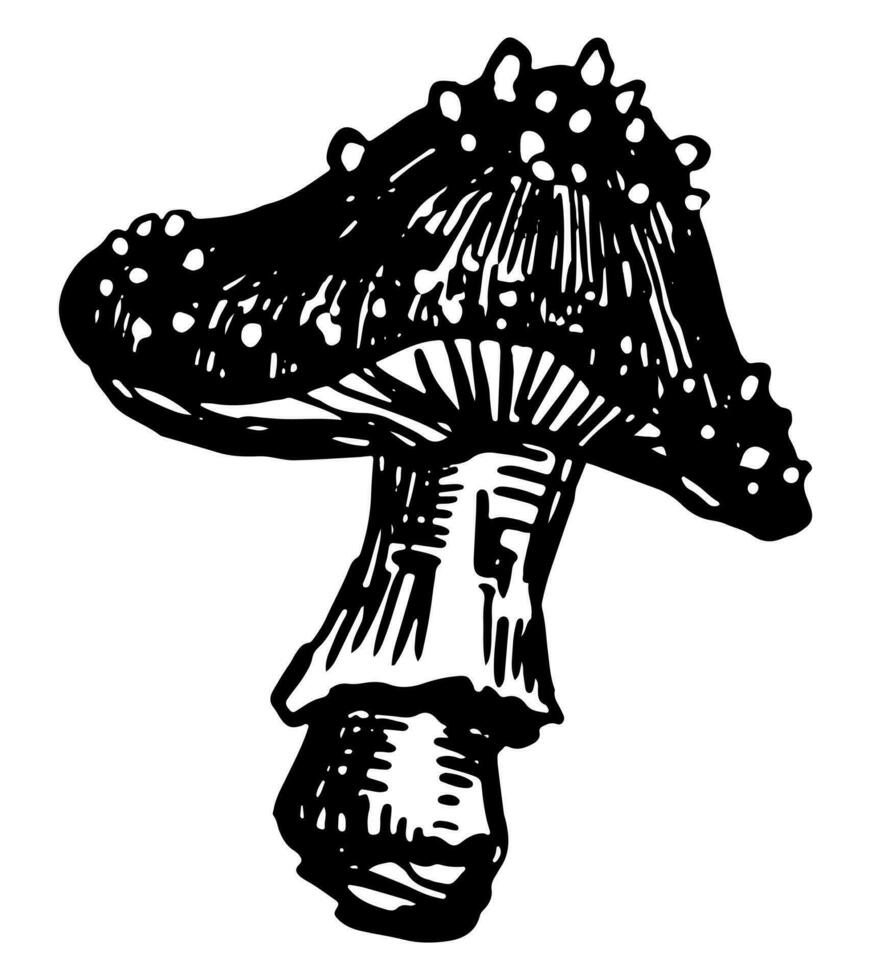The image is a black and white computer-generated drawing of a unique mushroom resembling a toadstool, reminiscent of fantastical settings such as those in a Willy Wonka story. The rough illustration, seemingly drawn with a black marker, features the mushroom's distinct stalk and cap. The underside of the cap showcases prominent striations, representing the gills. The cap itself is adorned with numerous wart-like protrusions, which are white circles outlined in black, giving it an unusual textured appearance. The background is stark white, emphasizing the details of this peculiar and somewhat unrefined mushroom drawing. The overall impression is that of a rough, monochrome sketch, focusing solely on the mushroom with no other elements present.